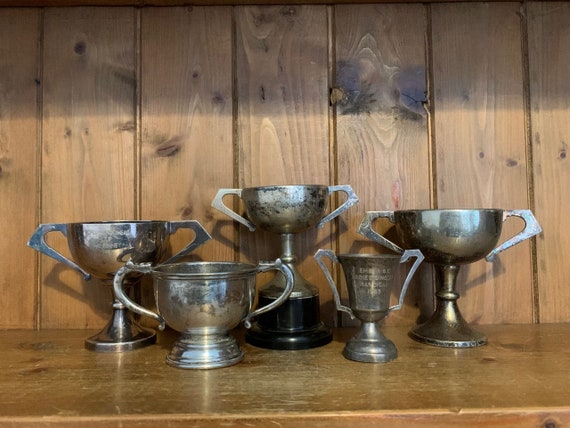The image depicts a collection of five tarnished silver trophies, arranged on a wooden shelf against a backdrop of wood paneling. The trophies, each featuring handles on both sides for easy lifting, vary in height and width, with the three tallest positioned at the back and the two shorter ones at the front. The central tall trophy in the back stands out with a distinctive black pedestal base, while the others rest entirely in their silver form. Although the inscriptions on some trophies are visible, they remain illegible due to the tarnish. The trophies' silver surfaces show signs of aging and neglect, with noticeable pitting that could be revitalized with a good polish.